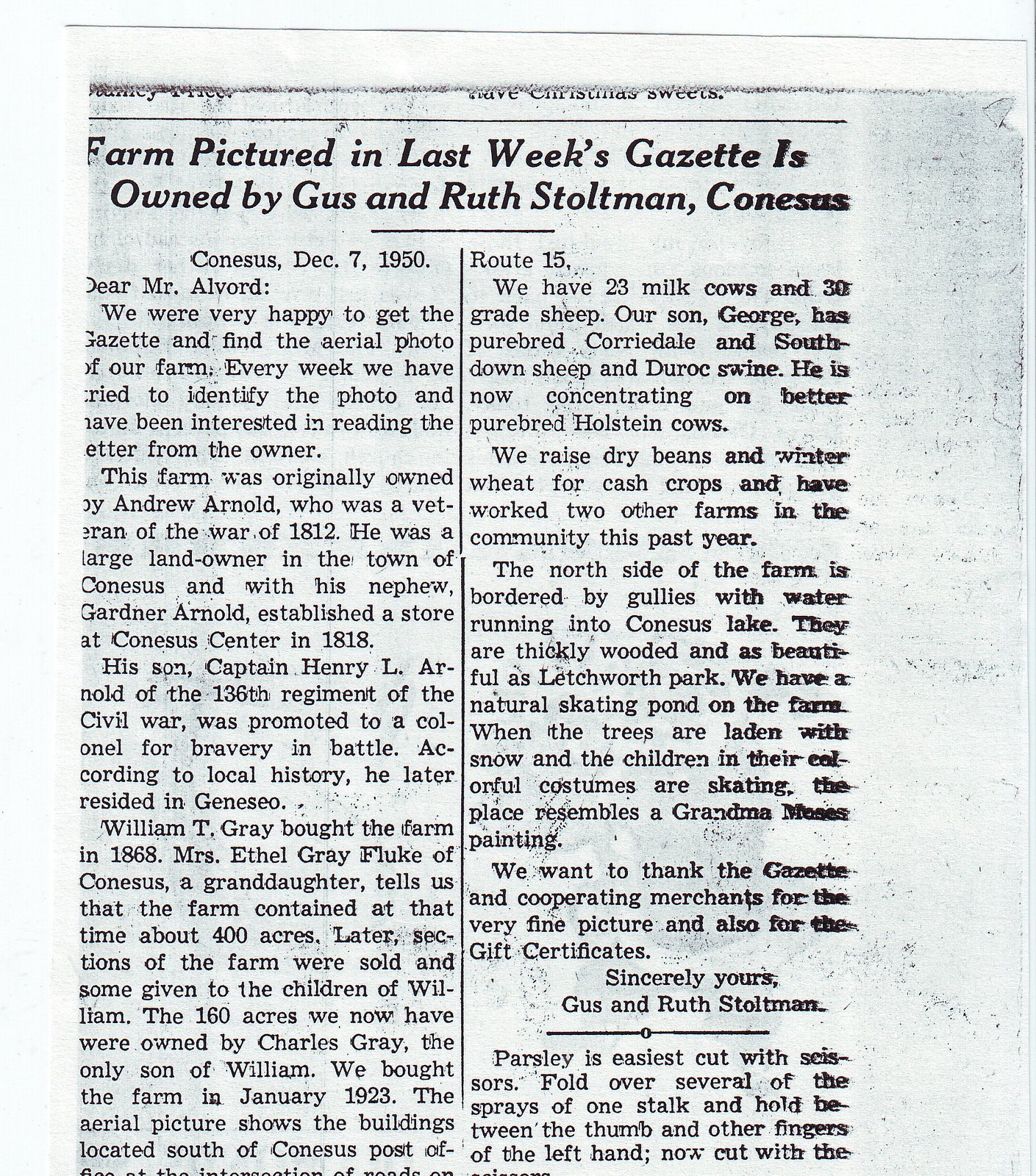This image is a scanned clipping of an old black-and-white newspaper article from December 7th, 1950, with the heading "Farm pictured in last week's Gazette is owned by Gus and Ruth Stoltman, Knesses." The article features two columns of text, with a slightly smeared right-hand side and minor tears at the top, indicating the age and wear of the original newspaper. The text begins with "Dear Mr. Alvord, we were very happy to get the Gazette and find the aerial photo of our farm," describing the Stoltmans' pleasure in seeing their farm featured. The letter details the farm's history, noting its original ownership by War of 1812 veteran Andrew Arnold and its subsequent ownership by various members of the Arnold family, including Civil War Colonel Henry L. Arnold. William T. Gray bought the farm in 1868, and according to his granddaughter, Mrs. Ethel Gray Fluke of Knesses, the farm spanned around 400 acres at that time. The letter concludes with "Sincerely Yours, Gus and Ruth Stoltman," with some additional text beneath. Despite the scans' imperfections, the article vividly portrays a significant piece of local history.